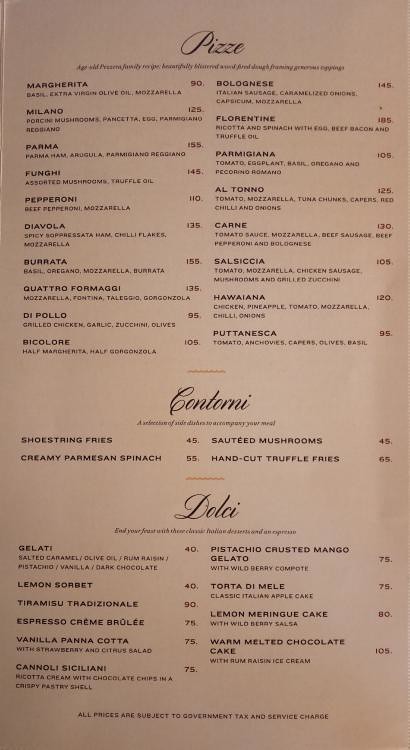The image depicts a slightly worn and unevenly folded menu from an Italian restaurant, printed on light brown paper with black text. The menu is organized into three sections. At the top is "PIZZE," listing various pizza options arranged in two columns, with offerings such as Margherita, Milano, Parma, Funghi, Pepperoni, Diavola, Burrata, Quattro Formaggi, Di Polo, Bicolore, Bolognese, Florentine, Parmigiana, Altono, Carne, Salsiccia, Bologna, and Purinesca. The prices for these pizzas range between 90 and 185 units. The middle section labeled "Contorni" features side dishes like shoestring fries, creamy Parmesan spinach, sautéed mushrooms, and hand-cut truffle fries, with prices between 45 and 65 units. At the bottom of the menu, the "Dolce" section offers desserts such as gelati, lemon sorbet, tiramisu, traditional espresso, crème brûlée, and melted chocolate cake, with prices spanning from 40 to 105 units. Despite the small, slightly hard-to-read text, the menu provides a clear and extensive selection of Italian delicacies.